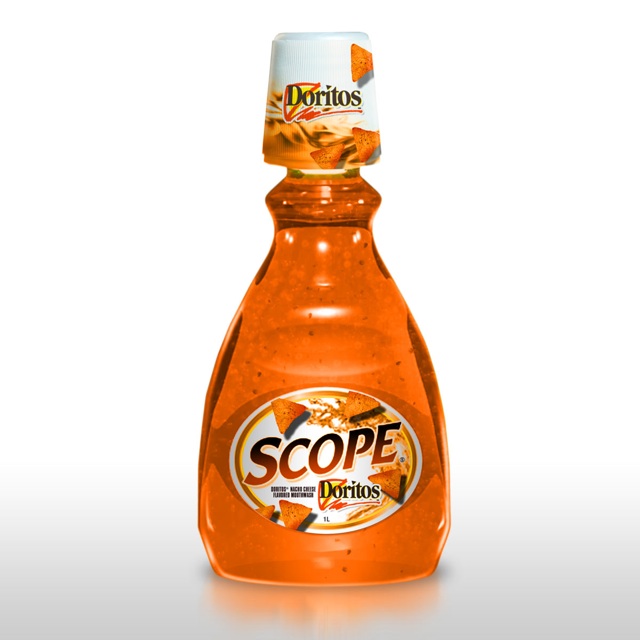In this vibrant color photograph, a bottle of Scope brand mouthwash takes center stage against a stark white background, ensuring all attention is focused on its intriguing features. The mouthwash inside the bottle is a striking orange color, indicating a unique variety. The bottle appears to have been opened, as evidenced by the absence of a plastic seal around the bottle cap, although the liquid level suggests it is still full.

The front label of the bottle is prominently displayed, drawing immediate attention with its vivid imagery and text. The label, oval in shape, features the brand name "Scope" in bold, orangey-red letters. Below the brand name, the word "Doritos" is emblazoned alongside the iconic yellow triangle Doritos logo, outlined in red. Surrounding the text are five individual Dorito chips, artistically arranged and visually enhanced by their bright orange coloration, dusted with chili and other seasonings.

Mirroring the thematic design, the bottle cap is also adorned with the Doritos branding. Three Dorito chip images encircle the cap, reinforcing the thematic collaboration between Scope and Doritos. The overall composition of this image is both visually striking and highly detailed, highlighting the captivating fusion of a mouthwash product with the unexpected and bold branding of Doritos.